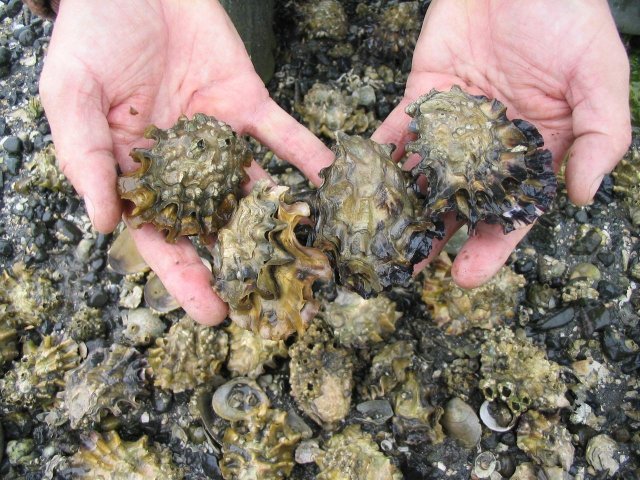The image captures a pair of hands, identified as belonging to a white person, reaching in from the top of the photo, palms upward, and holding four wavy, unoccupied shells that exhibit a blend of green, brown, and black colors with hints of gold. These shells, resembling mollusks or possibly oysters, are positioned prominently at the center of the photograph. Surrounding and underneath these hands, there is a dense bed of similarly colored shells, ranging from light brown at the base to darker brown and almost black towards the edges. The environment, filled with an array of these shells, remains ambiguous as to whether it is underwater or within a tank, but the shells visibly originate from a marine setting. The overall scene immerses the viewer in a detailed and textured depiction of marine life handled by human hands.